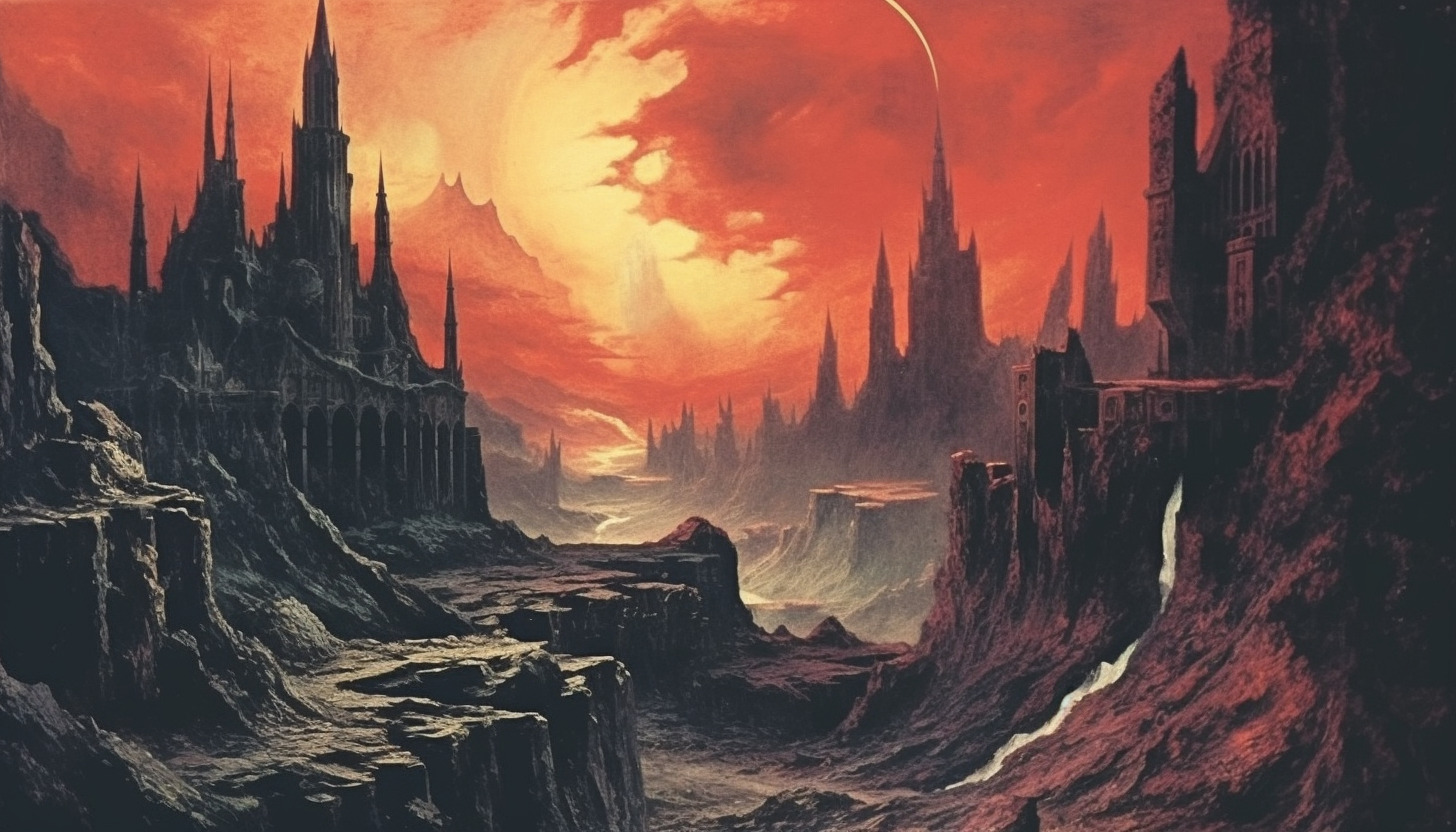This digital painting, evocative of a dystopian fantasy landscape, features a chaotic, rocky terrain dominated by hues of red, orange, yellow, brown, and black. The scene is devoid of any vegetation, contributing to its hellish atmosphere. To the left, a dilapidated castle is intricately built into a towering cliff, featuring multiple arches at its base and rising spires reaching up into a sky ablaze with red and yellow tones. The central area of the painting shows a winding valley extending from the lower bottom to the right center, then curving back to the left, with a small stream of water flowing through it. On the upper right side of the image, another castle emerges from the cliffside, its arched structure partly obscured but visibly worn. A diminutive waterfall cascades from beneath this castle, joining the stream in the valley below. The sky, heavily shrouded in ominous orange clouds, partially conceals what appears to be the sun, casting a surreal glow over the entire scene. The background is punctuated by additional spires and mountainous structures, enhancing the otherworldly, cavernous ambiance of the artwork.